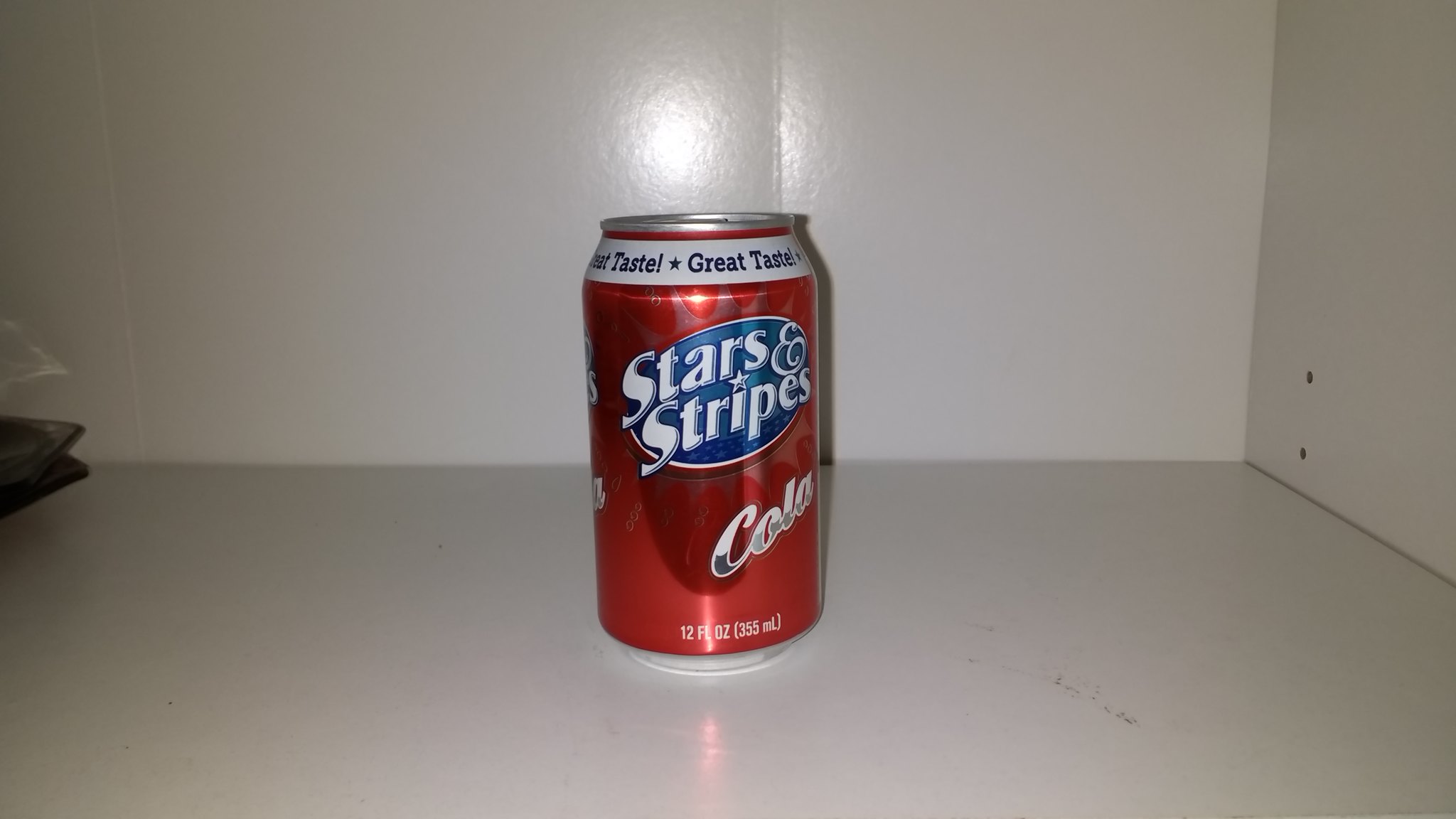The photograph captures a can of Stars and Stripes soda prominently positioned in the exact center of a pristine, white shelf. The background and surrounding side walls of the shelf are entirely white, ensuring all focus remains on the striking can. The can itself is vibrant, adorned in red, white, and blue colors. 

At the very top of the can is a silver band, immediately followed by a narrow band of red and then a white band inscribed with the phrase "Great Taste" accompanied by stars, appearing multiple times around the circumference. The main body of the can, which constitutes about 90% of its height, is predominantly red with silver accents. 

Front and center on this main body is a prominent blue oval that encompasses the brand name. The word "Stars" is written on the first line, followed by an ampersand and a star symbol in the middle, with "Stripes" written below. Underneath, the word "Cola" is displayed in white letters. 

Upon closer inspection, there appears to be something indiscernible on the shelf towards the center left of the image, but its exact nature remains unclear.